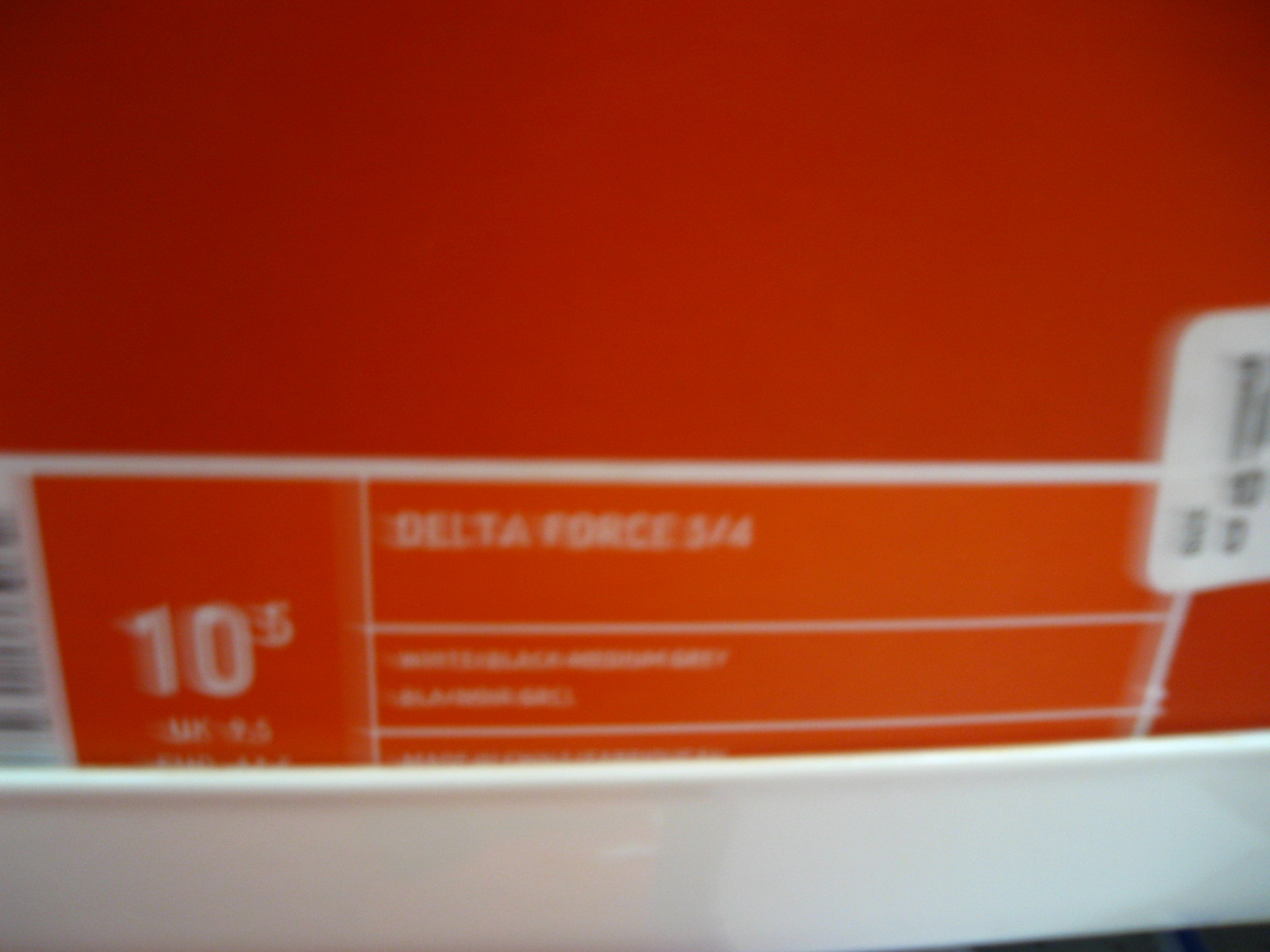This image is a photograph of an extremely blurred and poor quality close-up of an orange shoe box resting on a white metal shelf. The photograph focuses on the side label of the box, which makes it difficult to read specific details. At the top, the box is solid dark orange, transitioning to a lighter orange near the bottom with a white line separating the two shades. On the left side of the label, a partial barcode is visible, along with the shoe size stated as 10-1/2. In the middle of the label, the words "Delta Force" can be discerned, followed by "5/4" or "3/4." There is additional text beneath this, but it is too blurry to be read. In the right-hand corner, there is a white sticker with unreadable writing. The box appears to be placed in its white lid, adding another layer of white at the bottom of the image.